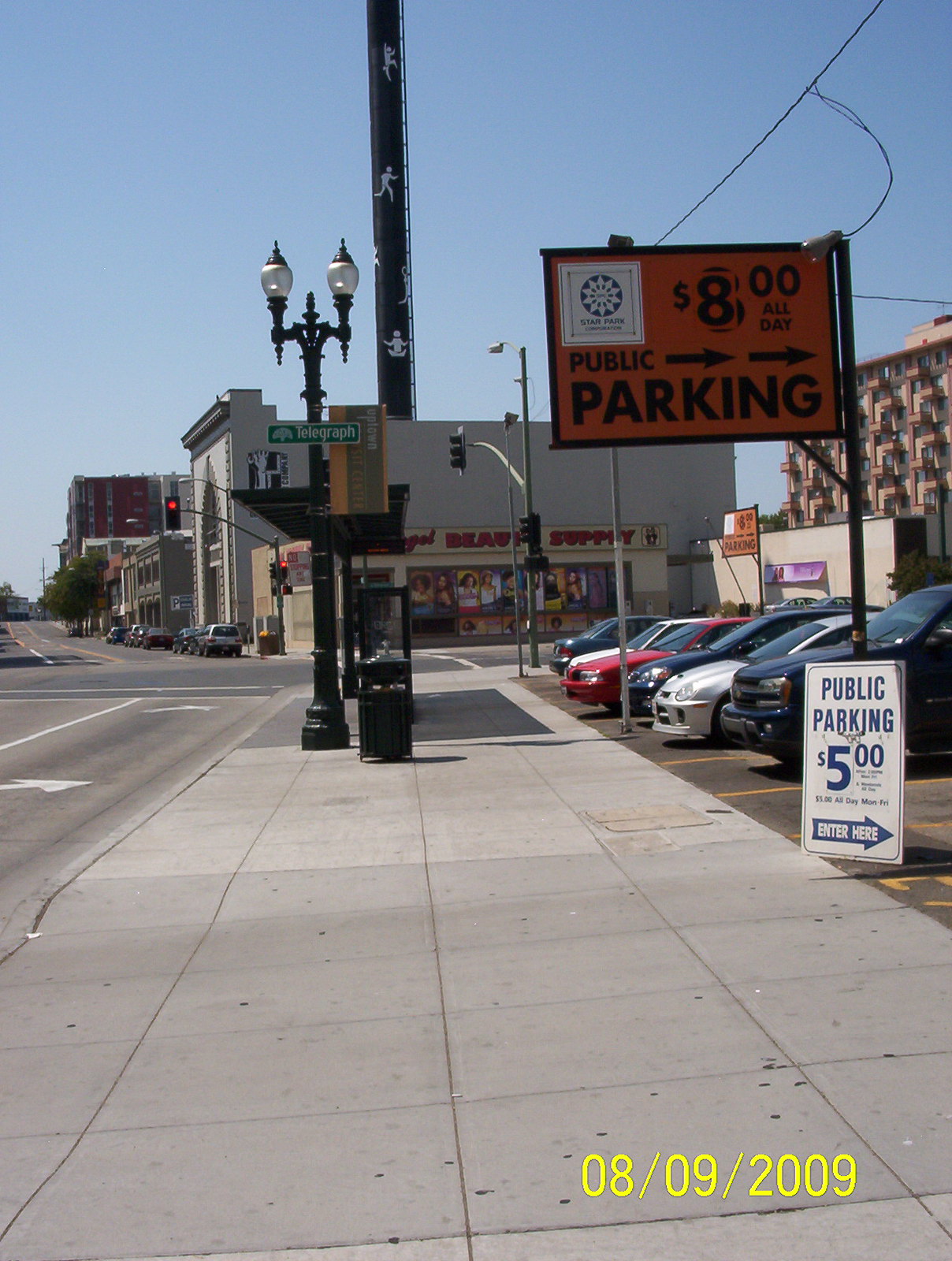The image depicts a detailed scene from a city sidewalk. The sidewalk is divided into large square tiles, arranged in a four-wide pattern, leading the viewer's eye down the path. Dominating the foreground is a tall, dark brown telephone pole adorned with white silhouettes of people engaged in various activities, such as walking and performing yoga poses. Adjacent to the pole is a vintage-style street lamp featuring dual lights and a horizontally-placed green sign with a white border that reads "Telegraph."

To the right of the image stands a vertical, rectangular sign, indicating public parking. It boldly states "Public Parking $5" in white lettering against a blue background, with a blue arrow pointing to the parking entrance. The sign further specifies "Enter Here, $5 All Day, Monday through Friday." Nearby, the entrance to the parking lot is marked by an orange sign, elevated on a tall pole, stating "Parking $8." This intricate setup provides an inviting yet bustling urban atmosphere.